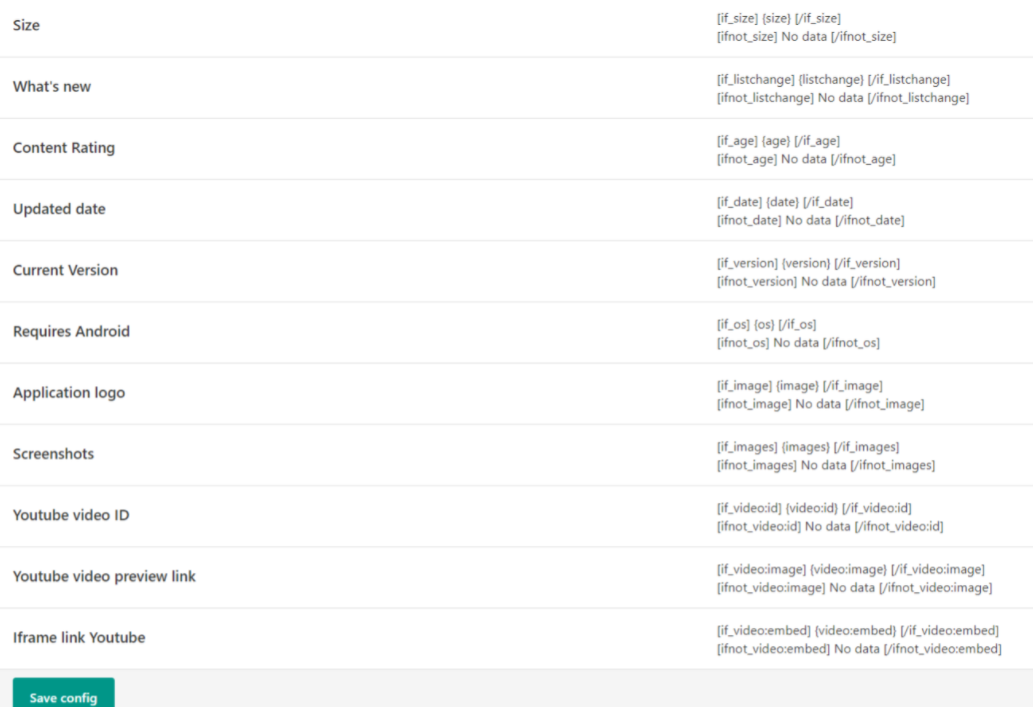This descriptive caption details a screenshot containing information about YouTube, presented in a structured layout:

---

The screenshot features a clean, white background with gray text. Starting at the top left, the heading "Size" is listed. Continuing down the left side, the following categories are detailed in order: Size, What's New, Content Rating, Updated Date, Current Version, Requires Android, Application Logo, Screenshots, YouTube Video ID, YouTube Video Preview Link, Iframe Link, and YouTube. At the very bottom left corner, there is a teal square button labeled "Save Config."

On the right-hand side of the screenshot, clickable links are displayed. Although the exact purpose of these links is not immediately clear, they appear as technical references or pathways to associated resources.

---

This comprehensive description encapsulates the layout and specific elements in the screenshot, providing a clear understanding of its content and organization.